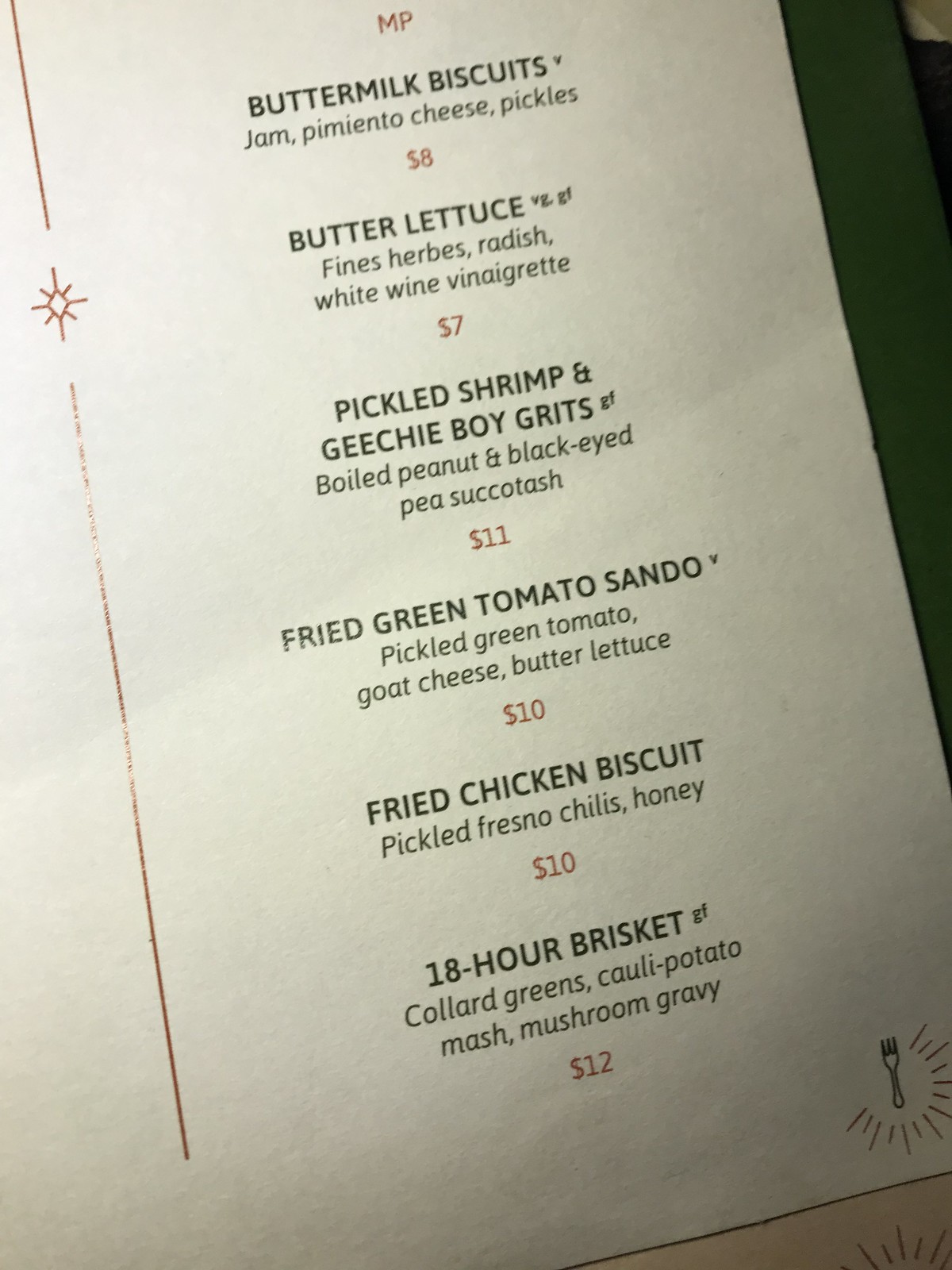This image captures a diagonally angled portion of a menu page, showcasing around 60-70% of its contents. The uncovered menu appears vulnerable to potential spills, requiring replacement in such an event. The menu layout is unconventional, lacking clear sections for appetizers, main courses, desserts, or other typical categories. All prices are included for each item. 

The top item is "Buttermilk Biscuits with Jam, Pimento Cheese, and Pickles" priced at $8. Following this is "Butter Lettuce," labeled VG for vegetarian and GF for gluten-free, with fine herbs, radish, and white wine vinaigrette, priced at $7. 

"Pickled Shrimp and Geechee Boy Grits," also gluten-free, is listed next along with "Boiled Peanut and Black-eyed Pea Succotash" costing $11. The menu includes a "Fried Green Tomato Sandow," possibly indicating a vegan or vegetarian option, with pickled green tomato, goat cheese, and butter lettuce for $10. A "Fried Chicken Biscuit with Pickled Fresno Chilies and Honey" is priced at $10. 

Lastly, the "18-hour Brisket," denoted as gluten-free, is served with collard greens, cauliflower potato mash, and mushroom gravy for $12. In the bottom right corner, the image features a clipart of a fork with various dashed lines emanating from it.